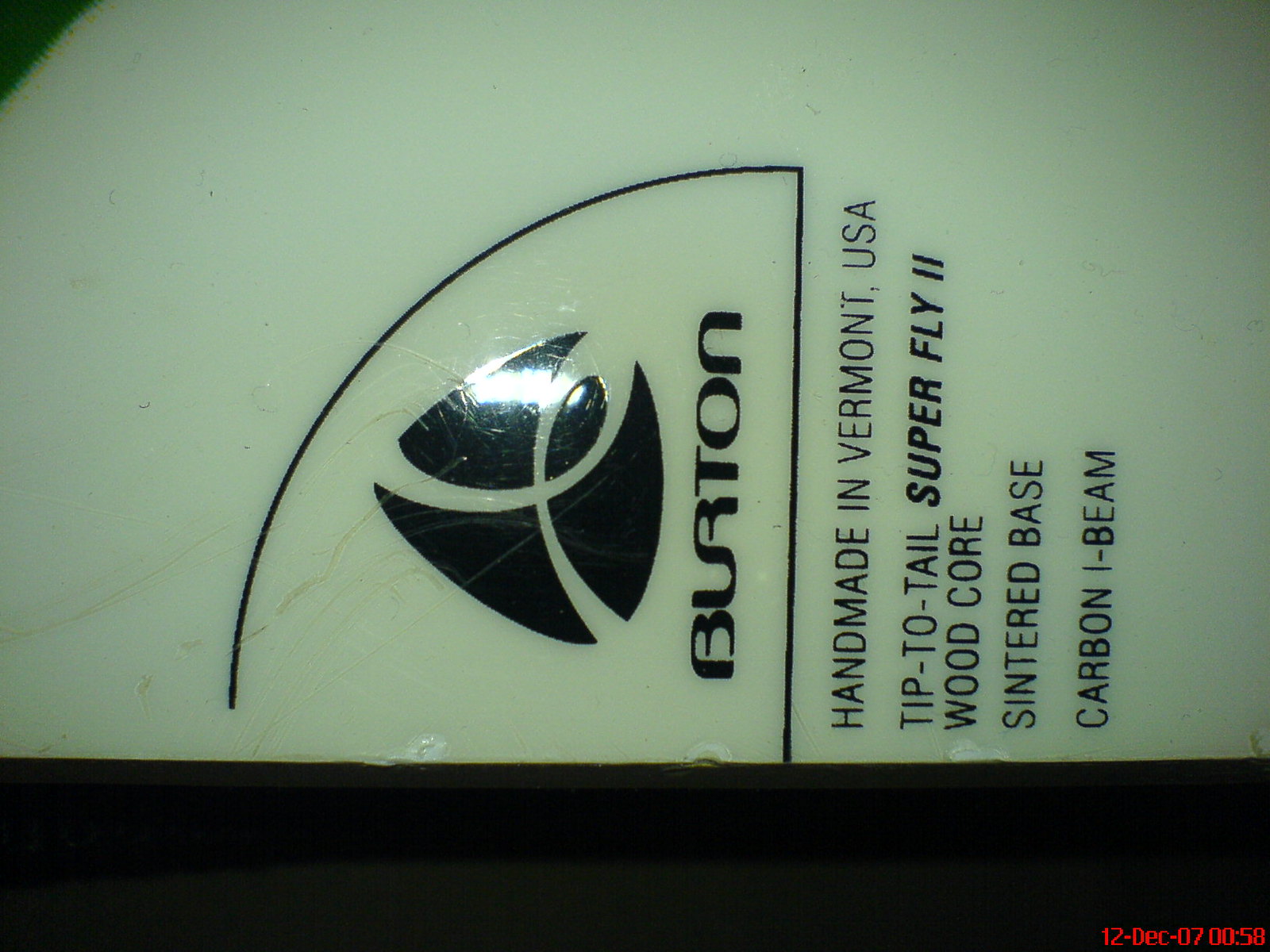This photograph features a graphic printed on a green, plastic-like material, captured in landscape mode with the text oriented vertically. A black bar runs beneath the item, which has a clear sticker adorned with black text. From bottom to top, the sticker reads: "Burton" in bold black font. Just above the Burton logo, there is a clear curly cue design on a black shield, revealing the green background beneath. Below the Burton logo, a black line divides the text, followed by the phrases “handmade in Vermont, USA," “tip to tail,” "Superfly II," "wood core," "sintered base," and "carbon beam," sequentially listed. The meticulous details in this caption add clarity and context to the visually complex image.